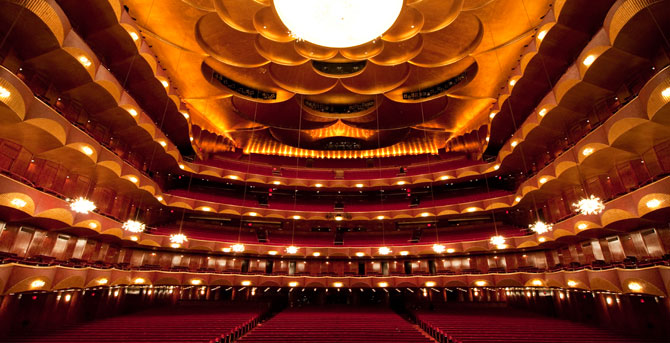A modern concert hall, likely the Baltimore Symphony Hall, is depicted in this image. The venue boasts striking post-modern and mid-century modern chandeliers, which circle elegantly around the space. The ceiling features artistically rounded sound panels designed to enhance the acoustics. The hall is bathed in a warm, yellow glow, creating a welcoming and vibrant atmosphere. Rows of red seats in front of the orchestra section add a touch of classic elegance to the contemporary design.